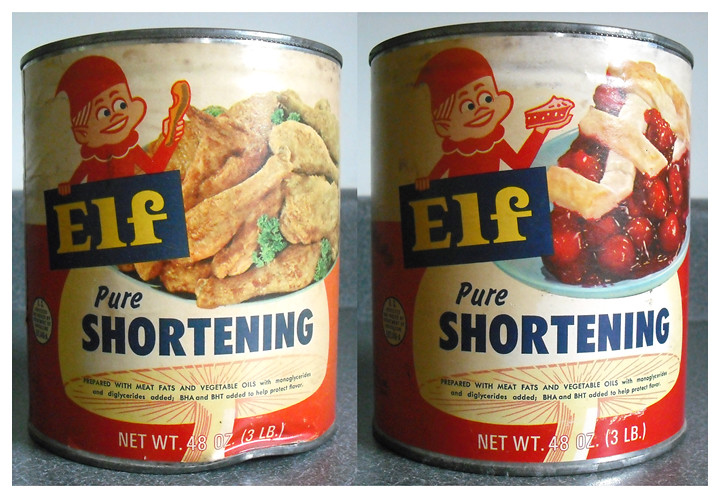The image shows two antique 48-ounce metal cans of Elf Pure Shortening, positioned side by side on a granite countertop with a light gray background. The labels, aged yet vibrant, prominently display red, dark blue, and yellow colors. Both cans feature a cartoon elf, with each can depicting different food items: one shows a realistic image of fried chicken and greens, paired with the elf holding a piece of fried chicken, while the other showcases a cherry pie, with the elf presenting a slice of pie. The label includes a navy blue rectangle banner with 'Elf' written in yellow letters. Additionally, both cans highlight "Pure Shortening" prepared with meat fats and vegetable oils below the respective food images.